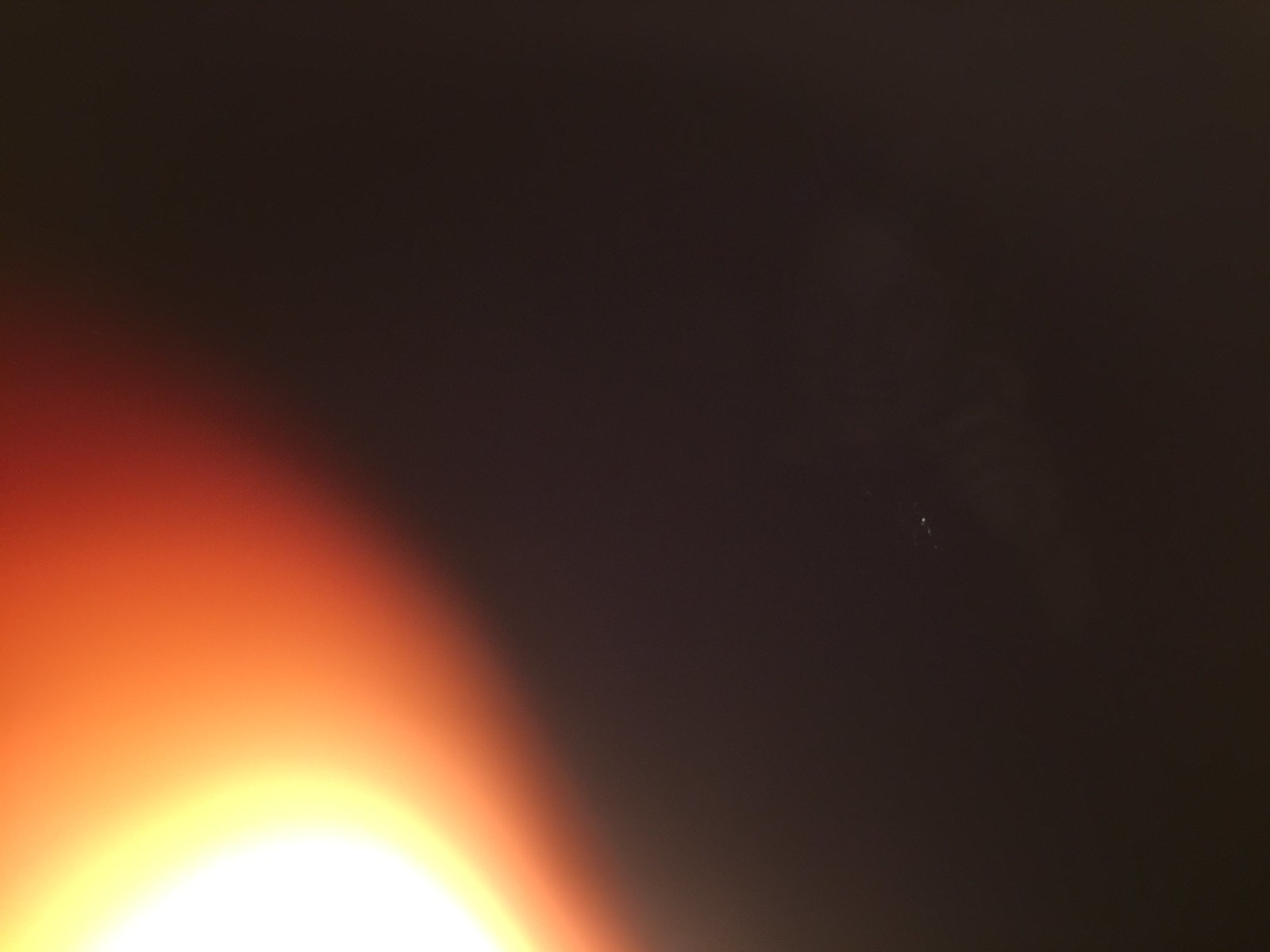The image predominantly features a dark, nearly black background. On the left side, there is a striking light source resembling a flame. At the very bottom left corner, a bright white light emerges, revealing about a quarter of a circle before it extends off the image's edge. Above this luminous white light, a vivid yellow line radiates upwards. This yellow hue then gradually transitions into a slightly darker shade infused with red and hints of gray. Continuing upward, the color shifts to a vibrant orange that deepens into a richer red as it ascends. At the top of this light source, there is a faint mist of pink. The remainder of the background remains in pitch darkness, accentuating the dramatic interplay of light and color on the left side.